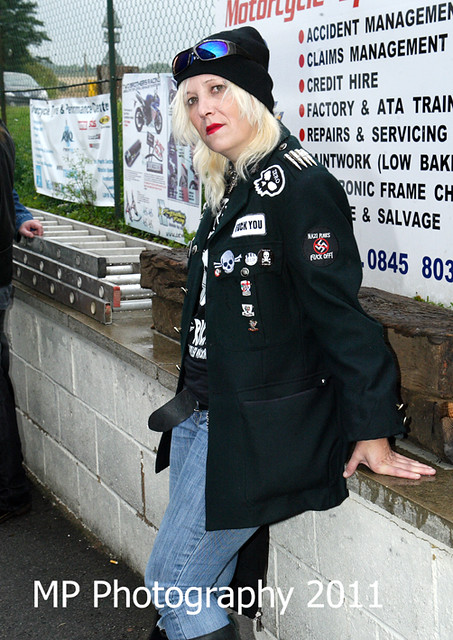An image captures a Caucasian woman leaning against a half wall made of white stone with a gray ledge on top. Attached to this wall is a chain-link fence and a banner hanging behind her. A silver ladder is visible in the background above the ledge. The woman, dressed in blue jeans and a long-sleeve black coat resembling a motorcycle jacket, has several badges and patches, including a skull and bones emblem and a circled swastika with a red line through it, indicating her disdain for Nazis. She also has "FU" on her left lapel. Underneath the coat, she wears a black and white shirt adorned with pins on the front. Her head accessory includes a black beanie, and she sports mirrored sunglasses. Her white-blonde hair and red lipstick complement her overall edgy appearance. The bottom of the image contains the text "MP Photography 2011."